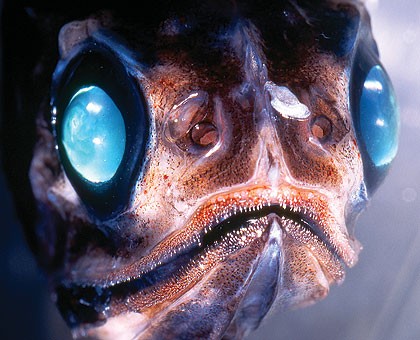The image features a close-up of the head of an exotic, deep-water fish with a notably ugly appearance. Dominating the fish's visage are its prominently large, turquoise blue eyes set wide apart, surrounded by dark, almost black patches. Between these eyes, the fish's nostrils are visible as two small holes on the nose ridge. The fish's mouth is mostly closed, revealing no obvious teeth but suggesting minor abrasions. Its skin appears slimy, predominantly light brown with patches of black, white, and orange, and it has a bony, lumpy texture. The background is blurred, likely water, fading out to ensure focus remains on the fish's intricate face. There is also a visible flat, solid triangle shape below its chin extending downward.